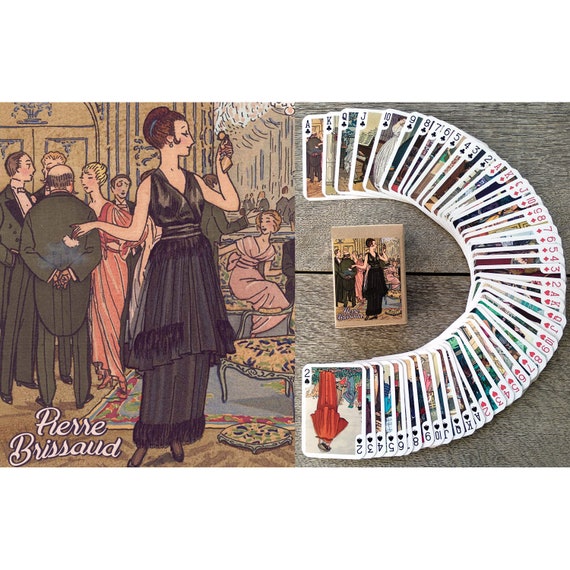The image showcases an elegant advertisement for a deck of customized playing cards. On the right side, the cards are spread out in a fan to reveal their diverse numbers and suits, starting from an ace down to a two. Each card features intricate artwork, consistent with the same high-end artistic theme. At the center of this fan of cards, the deck's packaging is prominently displayed. This packaging boasts a 1920s-style illustration resembling a high-society French scene, depicting a sophisticated woman in a black, sleeveless dress with an overlay skirt and black shoes. The woman, with her hair elegantly styled up, holds an object in her left hand while her right arm extends in a poised gesture. She appears to be at a glamorous party, surrounded by well-dressed figures in suits and gowns, reminiscent of a gala or ballroom setting. At the bottom left of the illustration, the name "Pierre Brassard" is inscribed, adding to the artwork’s refined and opulent feel.